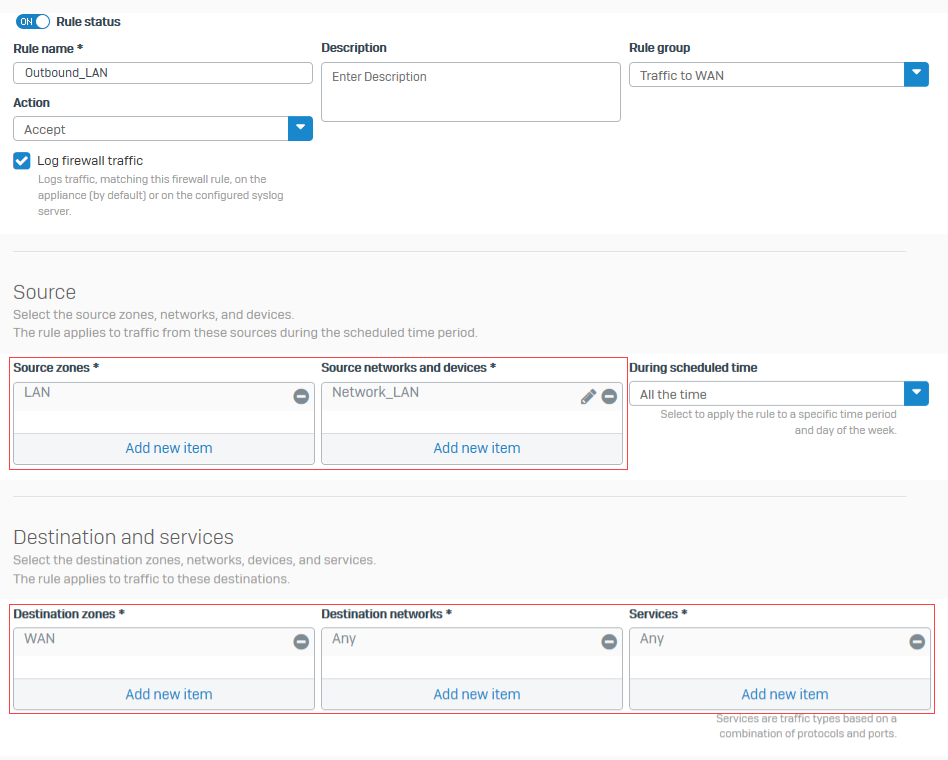The image appears to depict a section of a networking or firewall configuration webpage, specifically focused on setting up rules for traffic management. Here is a detailed description:

---

The webpage displays a detailed interface for configuring firewall rules. The section titled "Rule Status" indicates that the rule is currently active. The "Rule Name" field contains the identifier "outbound_LAN." 

In the "Description" field, users are prompted to enter a description for the rule. The "Rule Group" section features a drop-down menu, currently set to "Traffic to WAN."

The "Action" drop-down menu is set to "Accept," and this option is selected with a checkmark. There's an option labelled "Log Firewall Traffic," which logs traffic matching this firewall rule either on the appliance or the configured Syslog server.

"Source" configuration allows the selection of source zones, networks, and devices to which the rule applies. The "Source Zones" field is currently set to "LAN" but appears to be disabled. Similarly, the "Source Networks and Devices" field contains "network_LAN" and is also disabled.

The "Scheduled Time" field features a drop-down menu where "All the time" is currently selected, indicating the rule is active at all times.

---